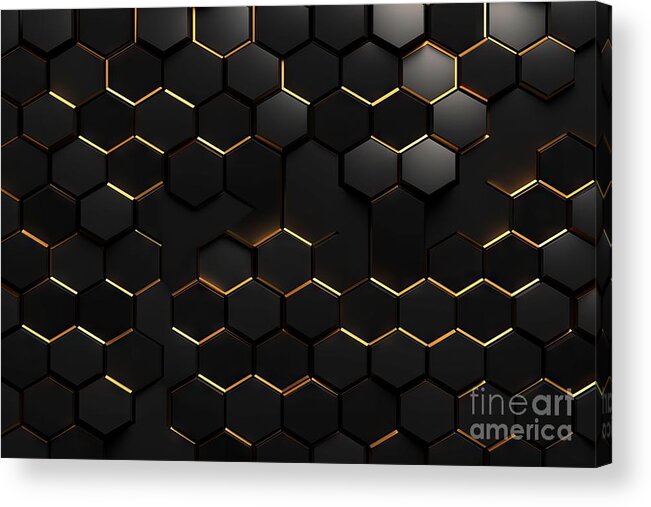This image features a striking and intricate mural design modeled after a honeycomb or beehive motif, prominently displaying hexagonal tiles arranged in rows. The tiles are predominantly black with golden-yellow outlines that accentuate their shapes, giving the design a discernible 3D effect. Some hexagons are slightly protruding while others appear recessed, adding depth and dimension to the overall artwork. Small, varying sizes of the hexagons and subtle differences in their protrusions enhance the visual complexity of the piece. The entire design is printed on canvas, and in the bottom right corner, there’s a Fine Art America logo, indicating the image's origin or affiliation. With its elegant yet simple composition, this image could serve as a sophisticated background for digital use or as a decorative element in various settings.